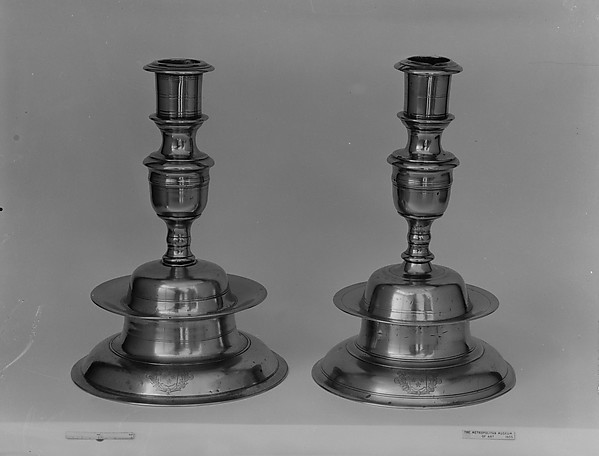This black-and-white photograph features two symmetrical antique silver candle holders set against a light gray, slightly curved background, appearing to rest on a similar gray surface. The candle holders are positioned centrally, side by side, but the one on the right seems slightly tilted compared to the more upright left one. The candle holders have an ornate, bell-like form with multiple circular layers and narrow at the top, resembling a wine cork, designed to fit a candle. Both items are highly reflective, though not in mint condition, with scuffs and dots indicating use. They feature intricate engravings near the bottom, possibly depicting small emblems like a little dog. The left candle holder seems to be missing a small circular knob present on the right. Small unreadable labels lie beneath each holder. Despite minor imperfections, they exhibit a vintage charm and elaborate craftsmanship.